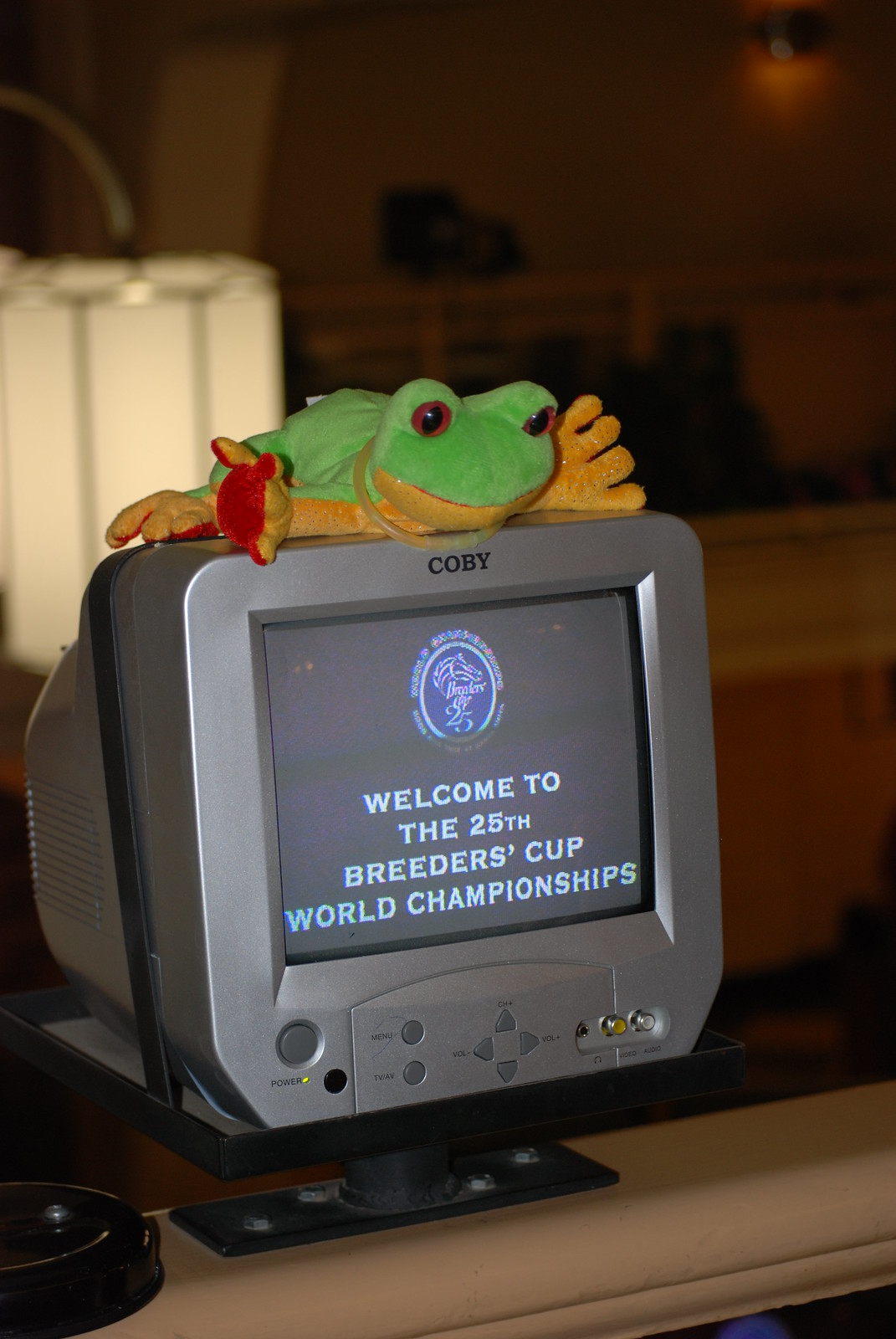The photograph, taken indoors and vertically oriented, showcases a quirky scene centered on a small, tube-style gray TV set by the brand Coby. Bolted to a light tan railing, the television screen displays the message, "Welcome to the 25th Breeders' Cup World Championship," accompanied by a blue circle with a horse head logo. Sitting atop this vintage TV is a charming, small stuffed frog reminiscent of a Beanie Baby. The frog features a green top with gold underbelly, hands, and feet, vertical brown eyes with black pupils, and it wears a gold necklace. The background is a blur of white and tan hues, possibly from a lamp or other indoor features, adding to the nostalgic ambiance of the setting. Beneath the TV, you can glimpse buttons for channel changing—both round and triangular—and a circular power button situated on the left side. A potential black ashtray is seen on the railing’s lower left corner, hinting at the indoor environment's casual, lived-in feel.